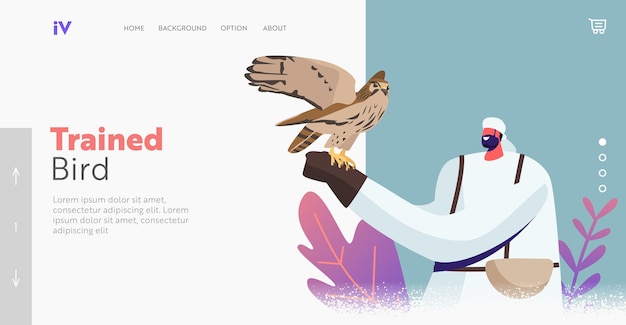The image is a computer screenshot of a webpage, likely an advertisement for a trained bird. In the upper left corner of the screen, it features the Roman numeral 'IV' in blue, followed by navigational tabs labeled "Home," "Background," "Options," and "About" in black text. On the far right, there is a shopping cart icon. At the middle left, the text "Trained bird" is prominently displayed, with "Trained" in red and "bird" in black.

The right side of the image showcases a cartoon graphic of a man dressed in white, wearing a turban and smiling, with a beard. The background behind the man is light blue. The man has his left arm extended, wearing a protective glove on which a brown falcon with yellow talons has landed. Additional details include gray navigation arrows pointing up and down located in the lower left corner.

Overall, the webpage presents a stylized and simplistic design, with elements of the text either unreadable or written in another language.